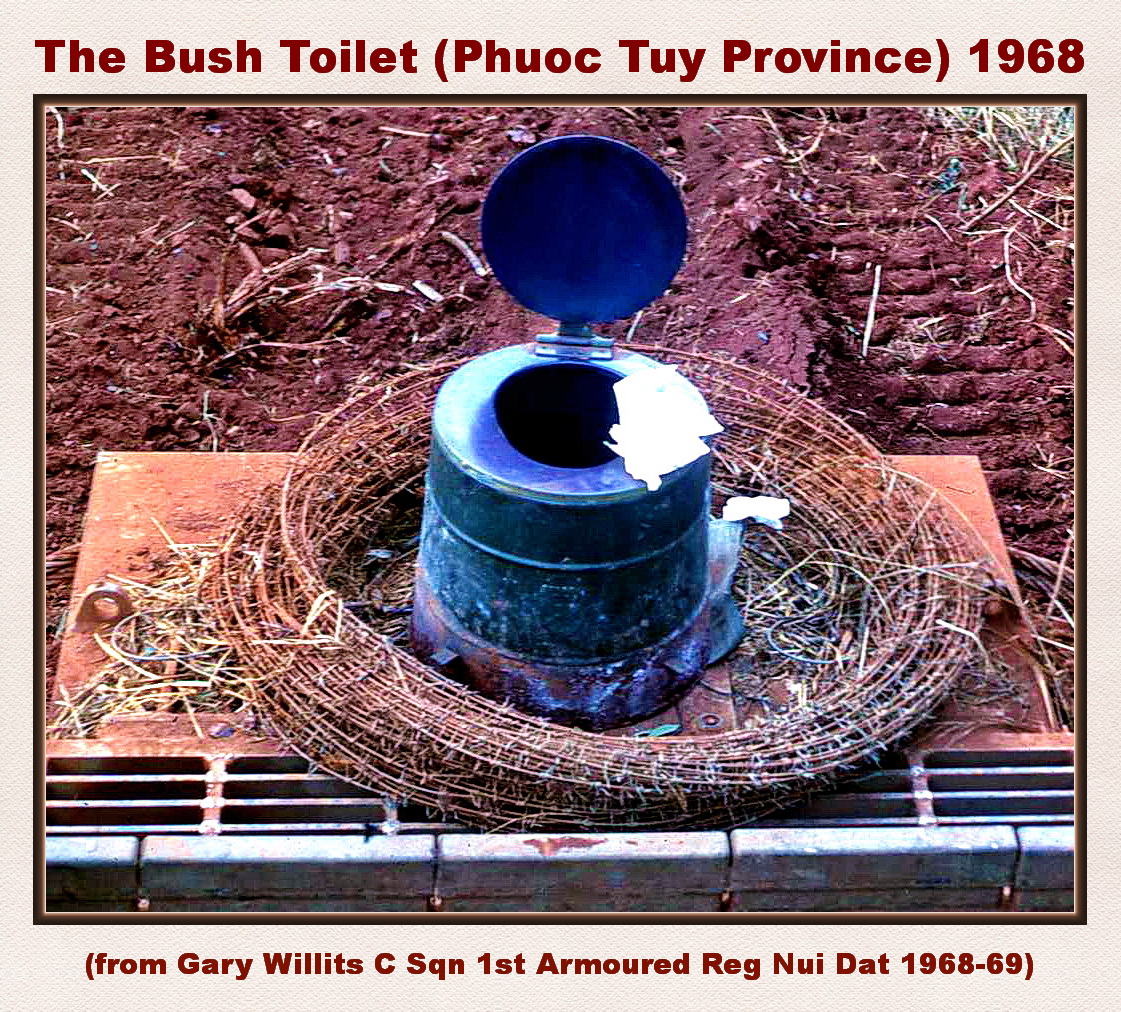The image is a historical photograph titled "The Bush Toilet, Phuoc Tuy Province, 1968." The photo is framed by a tan textured border with a dark brown inner line, resembling a picture frame. At the top of the tan border, in red font, reads "The Bush Toilet (Phuoc Tuy Province)" and "1968." At the bottom, it states, "(from Gary Willett's C-Squadron, 1st Armored Regiment, Nui Dat, 1968-69)." The central image features a rudimentary toilet composed of a bucket with a hole cut out and some toilet paper placed on top. This makeshift toilet is situated in what appears to be a nest-like structure, possibly made of wire and hay, indicative of field conditions typical of the Vietnam War era. The setting behind the bucket seems muddy, reinforcing the rugged environment. This photograph captures a functional yet primitive sanitation solution used by soldiers in the fields during the 1960s.